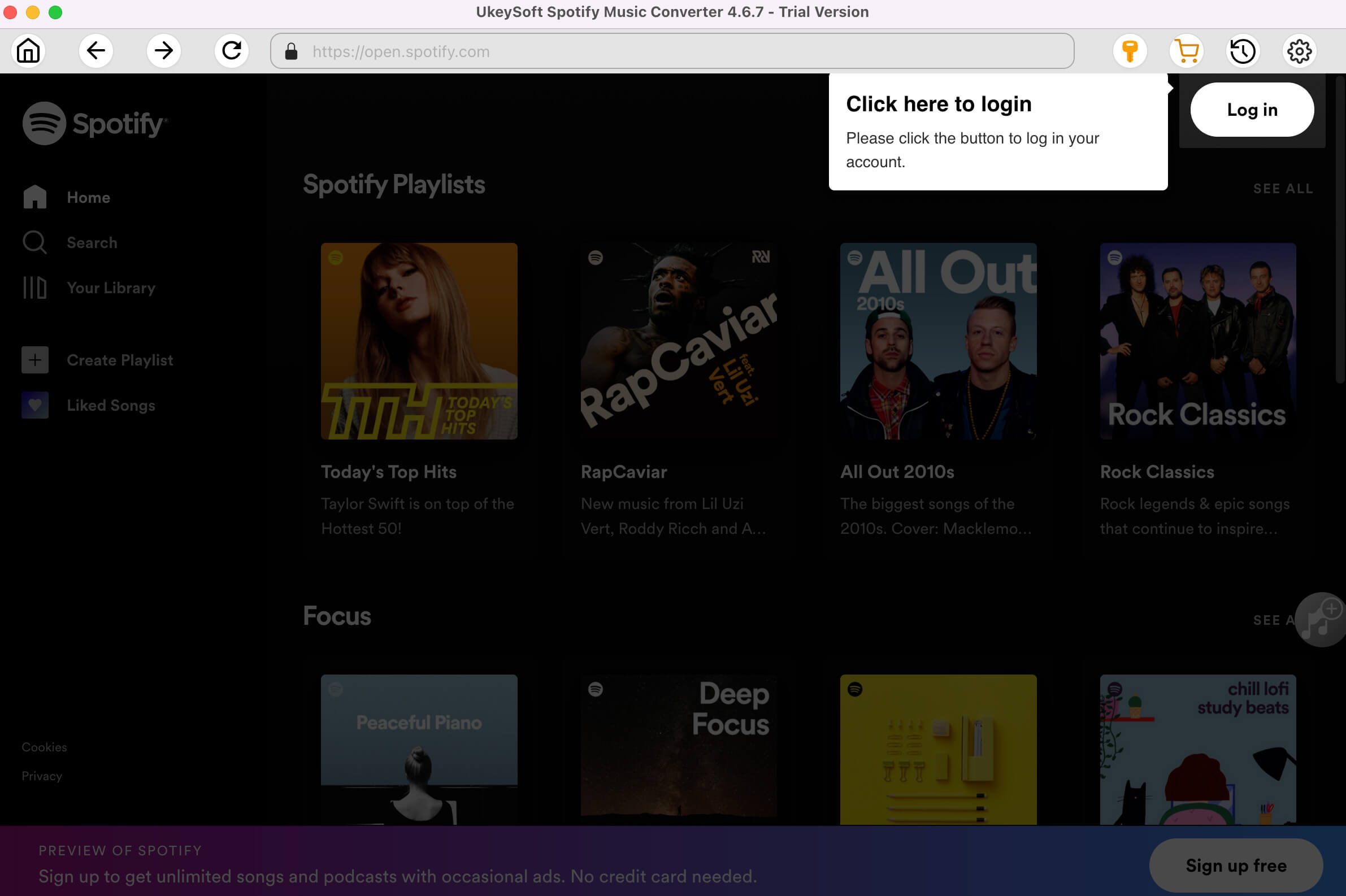The image showcases a screenshot of the Spotify web page. In the upper left-hand corner, there is the Spotify logo featuring three small horizontal black lines encased within a circle on a white background. Above this, a banner indicates the use of Ukeysoft Spotify Music Converter, version 4.6.7, marked as a trial version.

At the top of the interface, a series of navigational and functional icons are present: a home icon on the far left, followed by left and right directional arrows, a reload arrow, and a search bar. Additionally, there are icons for key functionalities: a key icon, a shopping cart icon, a clock icon signifying time-related functions, and a settings icon.

In the center of the page, a prominent message reads "Click here to log in," inviting users to log into their Spotify account by clicking the provided button within the shopping cart section.

The top left corner of the browser window features the classic three circular dots in red, yellow, and green, commonly associated with window control buttons for closing, minimizing, and maximizing the window respectively.

Lastly, the main content displays a special Spotify playlist, with a dedicated section below labeled "Focus," likely showcasing playlists or tracks designed to aid concentration or productivity.